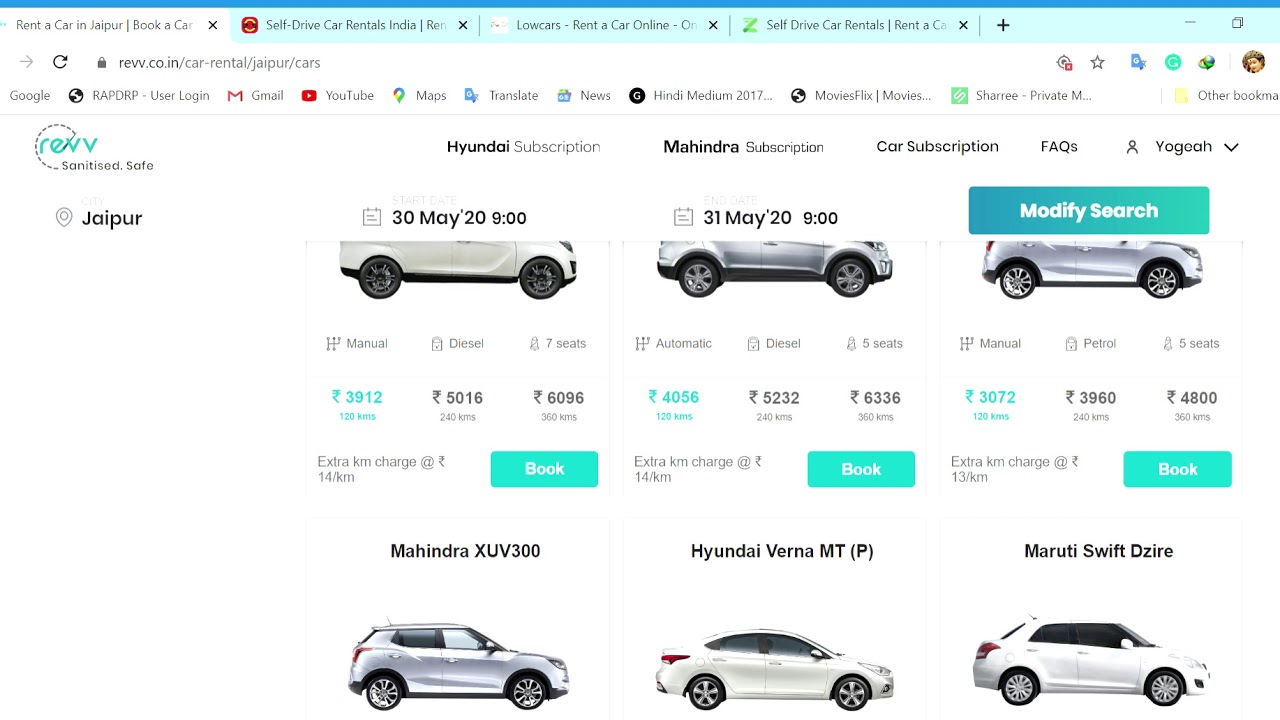**Screenshot Description**

The screenshot depicts a webpage showcasing various cars available for rental in Jaipur, India. The page is structured with a dark blue bezel at the top, below which multiple tabs are displayed. The selected tab, highlighted in white with black text, reads "Rent a Car in JAIPUR" (erroneously spelled as "Japer"), followed by the text "Book a Car" which is cut off, alongside an "X" symbol to close the tab. 

Beneath this is a red tab featuring a maroon red circle with two white bands, accompanied by black text on a cyan blue background that reads "Self-Driving Car Rentals in India." Adjacent to it, a white circle displays the text "Low Cars, Rent a Car Online" on a cyan blue background. Following that, a green square shows the text "Self-Drive Car Rentals." Situated on the right side of the page are collapse and window icons.

On the left-hand side of the page, a right-pointing gray arrow and a black refresh symbol are visible, next to a URL bar containing a dark gray padlock icon and the URL "revv.co.in/car-rental/jaipur/cars" in dark gray text. Below this, in light gray text, is "Google," followed by a black earth icon. In black text, the word "RAPDPVRP" is displayed alongside options to login, as well as symbols for Gmail (a red envelope), YouTube (a red square with a white triangle), Maps (a multi-colored pin transitioning from yellow to red to blue to green), Translate (a blue and white square), and News. Further listed are a circle with a "G" and "HINDI" text, a world icon labeled "Movie Fix Movies," and a green square with text cut off which reads "Sherry, Private...". Another yellow square labeled "Other Bookmarks" is partially visible and cut off.

The company logo at the bottom features a black dotted circle with teal letters spelling "REVV" and the words "Sanitize Safe" underneath it. Below this, the page highlights numerous cars for rental, available in various colors including silver, white, and dark gray, all priced in Indian rupees.